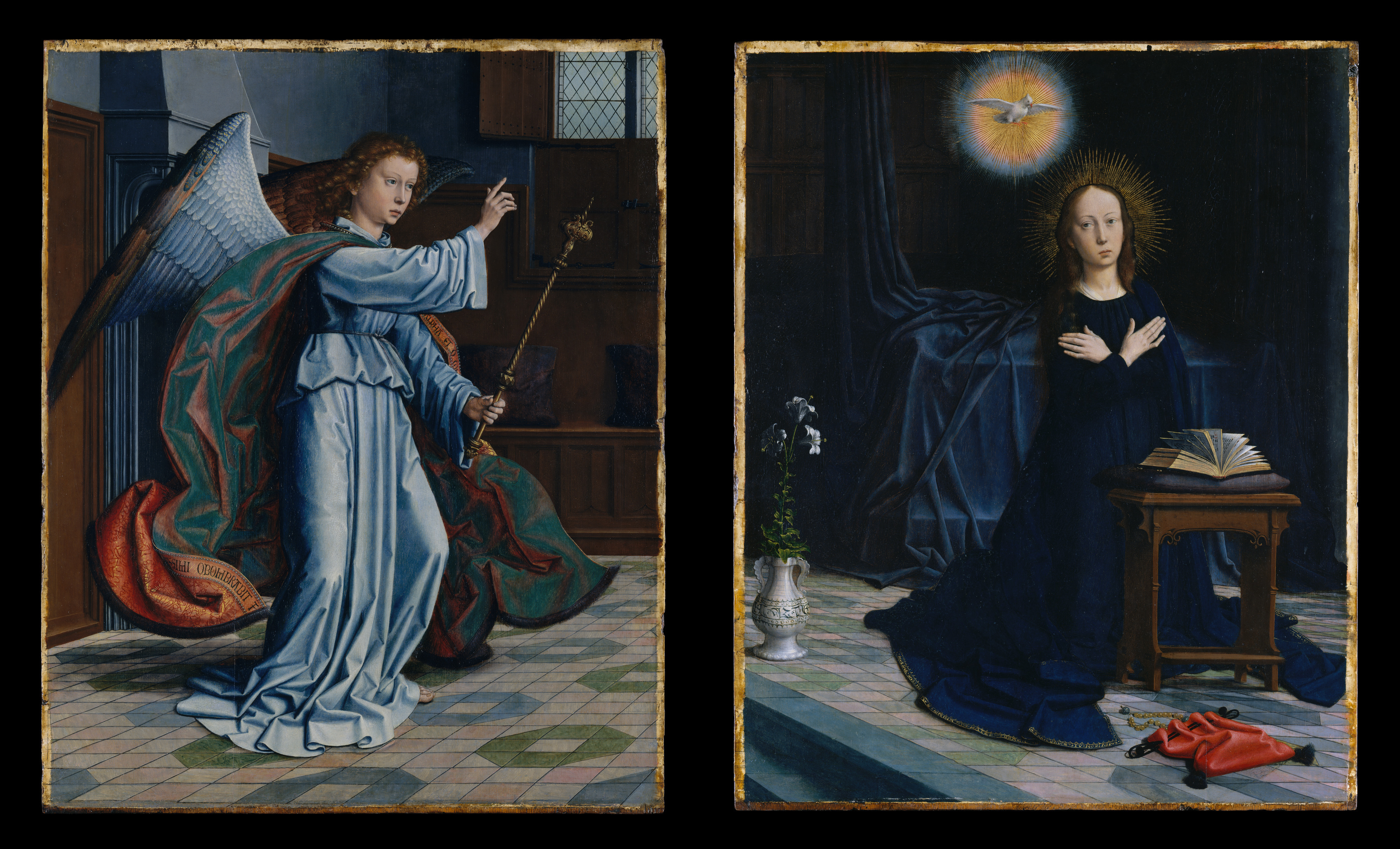The image showcases two side-by-side paintings, each framed in gold and set against a black background. Both paintings feature a religious theme and depict what appears to be the same female angelic figure in different settings. 

In the left painting, the angel is garbed in a long, silky blue robe with matching wings. She wears a large cape that is green and red and holds a golden, intricately designed staff in her left hand. Her right hand is raised, and she stands on a floor adorned with green and blue hexagon-shaped tiles.

In the right painting, the angel, now kneeling, wears a dark blue gown that extends to the floor. Her arms are crossed in front of her chest, and she kneels at a table draped in blue with an open book resting on a gray cushion. Above her, a circular stained glass window features a yellow sun with a white dove at its center. On the floor to the bottom right lies a red drawstring bag.